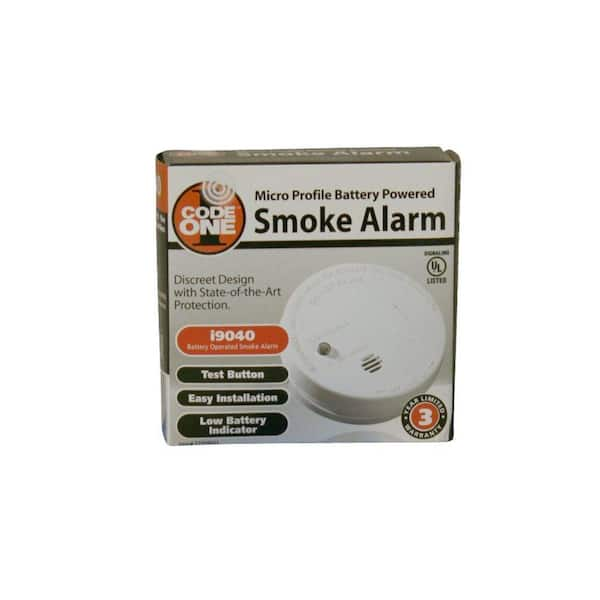This image showcases a product box for a smoke alarm against a white background. The box has a white, gray, and orange color scheme with detailed prints on the front. At the top, bold text reads "Micro Profile Battery Powered Smoke Alarm." Adjacent to this, there’s a logo featuring an orange circle with a black "1" inside, labeled "Code 1" in white text. Below this, there’s a photograph of a white, round smoke alarm, equipped with a small black speaker part on the lower left and a button in the middle. To the left of the photo, the text highlights features such as "Discrete Design with State of the Art Protection." Further down, the box describes additional functionalities, including "Test Button," "Easy Installation," "Low Battery Indicator," and specifies the "I9040 Battery." The bottom right corner of the box notes a "Limited Three-Year Warranty." The overall design suggests a modern, yet simple, aesthetic for this smoke alarm's packaging.